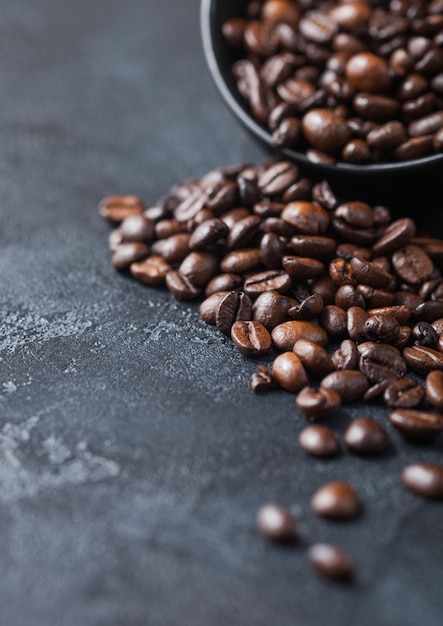The photograph captures an up-close scene of a black ceramic bowl, tilted at an angle, spilling an array of coffee beans onto a dark gray, textured surface that resembles a concrete floor. The beans, which are glossy and vary in rich shades of dark brown, are scattered in a small pile with a few stragglers farther away, suggesting they may have been dropped. The floor, in mostly dark gray with specks of light gray, enhances the contrast of the dark shiny coffee beans. The bowl, partially shown in the upper right corner, adds a dynamic element to the composition, emphasizing the motion of the beans spilling out and the tactile texture of the scene. The primary colors in this photograph are deep browns, black, and gray.